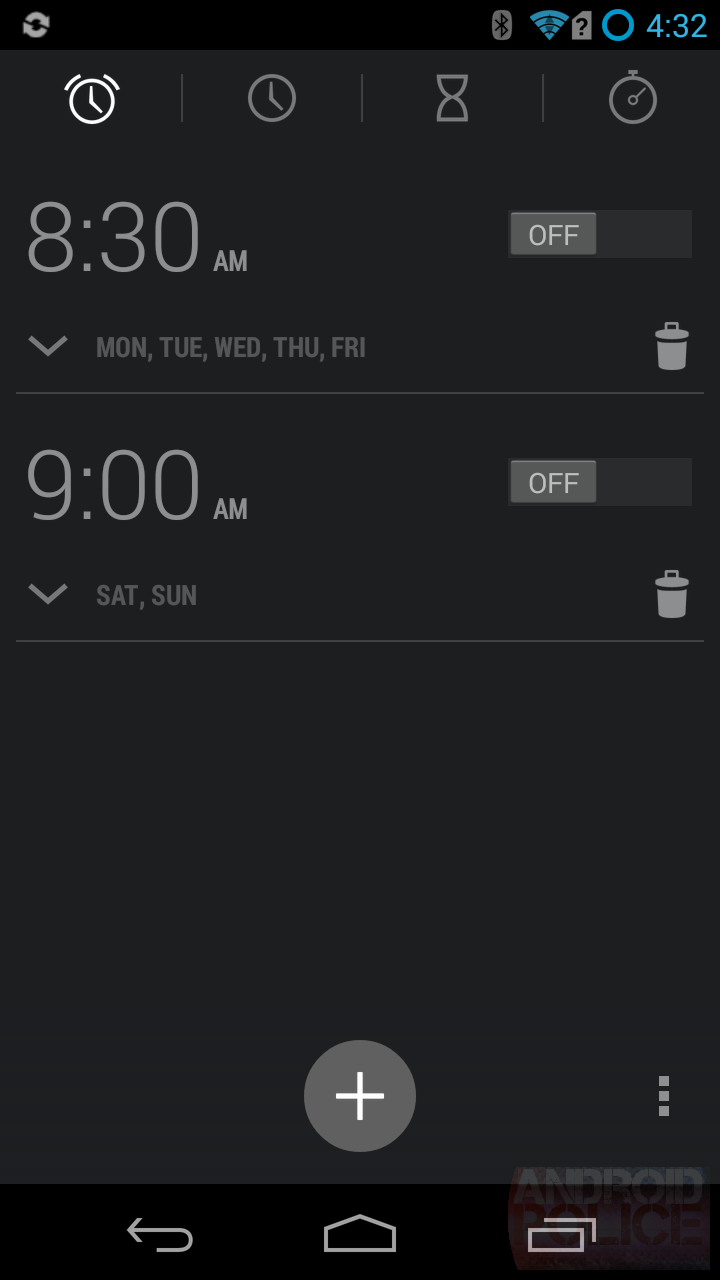Here is the cleaned-up and detailed caption for the image:

---

A close-up screenshot from an Android cell phone showing the alarm settings interface, set against a solid black background. In the top right corner, status icons for Bluetooth and Wi-Fi are visible, alongside a small box containing a question mark and a blue "O." The display reads "432" in blue.

The alarm configuration includes two separate settings:
- The first alarm time is set for **8:30 AM** on weekdays (Monday, Tuesday, Wednesday, Thursday, and Friday). Below the time, the abbreviated days "MUN, 2, WED, THU, FRI" are listed in gray text, with an arrow pointing down beneath the '8:30 AM' time. A gray box labeled "off" in white text and a gray trashcan icon are adjacent to this setting.
- The second alarm time is set for **9:00 AM** on weekends (Saturday and Sunday). Below this time, the abbreviated days "SAT, SUN" are listed in gray text, also accompanied by an arrow pointing down. This setting also has a gray box labeled "off" and a gray trashcan icon.

At the bottom of the interface, there is a gray circle featuring a white plus sign, indicating an option to add a new alarm. The screen clearly identifies the device as an Android phone, with the word "Android" appearing in the bottom right corner.

---

This rewritten caption provides a clean, detailed, and organized description of the image consistent with formal documentation styles.